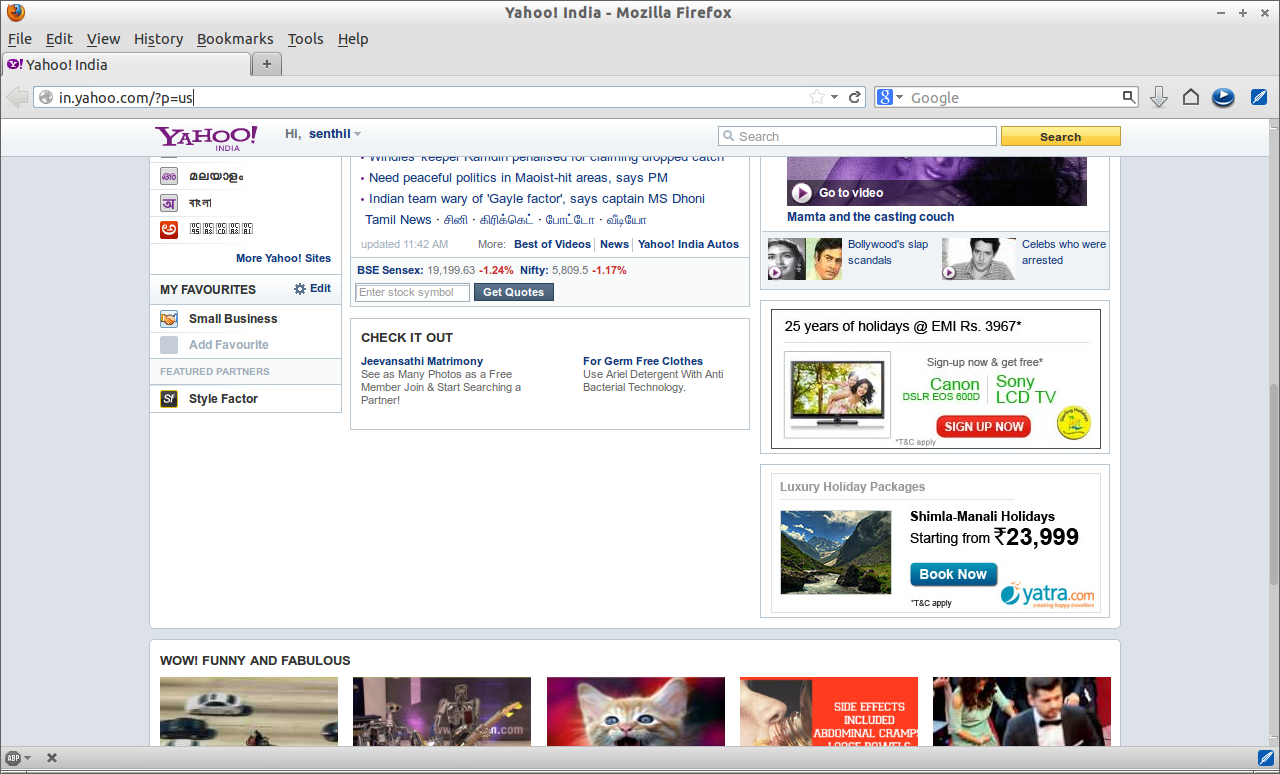Screenshot of Yahoo India webpage. At the top, the URL bar contains "im.yahoo.com/?p=US." The Yahoo India logo is prominently displayed below the URL. The page greets the user with "Hi Senphil," indicating the owner's account. To the left-hand side, various navigation options are available but presented in another language. A "My Favorites" section is visible, listing categories such as "Small Business." The "Featured Partners" section includes "Style Factor." In the center of the screen, several headlines are visible, some in English, including: "Need Peaceful Politics in Maoist-hit Areas, says PM" and "Indian Team Wary of Gale Factor, says Captain MS Dhoni." Other headlines and content appear in an unspecified language. Additional options for more content categories like "Best of Videos," "News," "Yahoo India Autos," are also present.